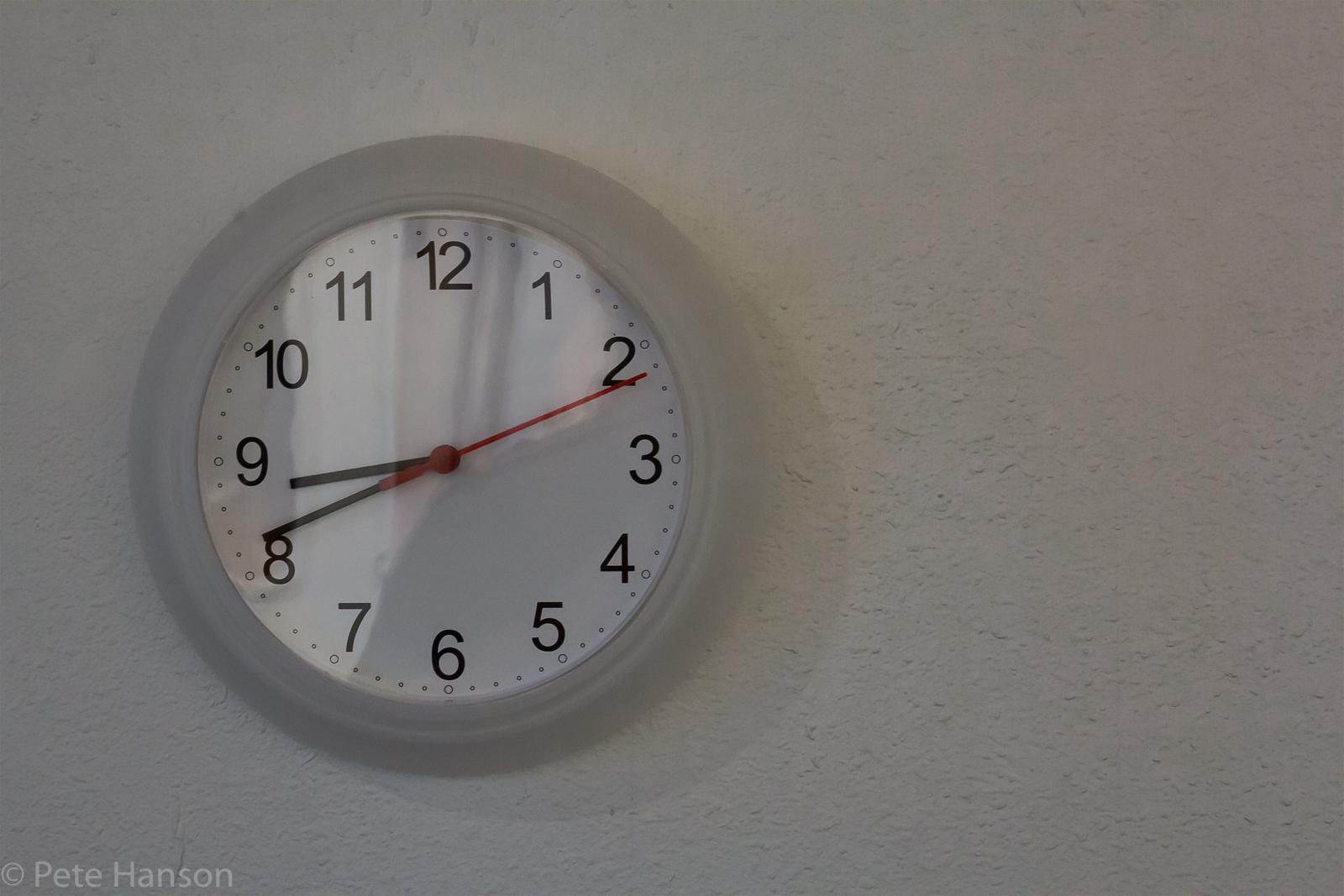A detailed photograph captures a clock mounted on a light gray, somewhat textured wall typical of institutional settings. The paint is not quite as thick as stucco but features a bumpier texture with subtle horizontal lines. In the left-hand corner of the image, there is a small watermark or signature that reads "C, circle, Pete Hanson." 

The rectangular image, oriented horizontally, places the clock on the left-hand side. The clock itself is framed with a light gray rim that encircles a white face displaying numbers from one to twelve, interspersed with small dots and four additional minute-indicating dots. Each hour mark features an added detail resembling a donut—numbers enclosed within small circles.

The clock's hands are black, with the hour and minute hands indicating 8:42. A red second hand is precisely at the 12 o'clock position. A glass or plastic covering protects the clock face and catches some light, resulting in reflections visible at the top and along the left edge of the clock.